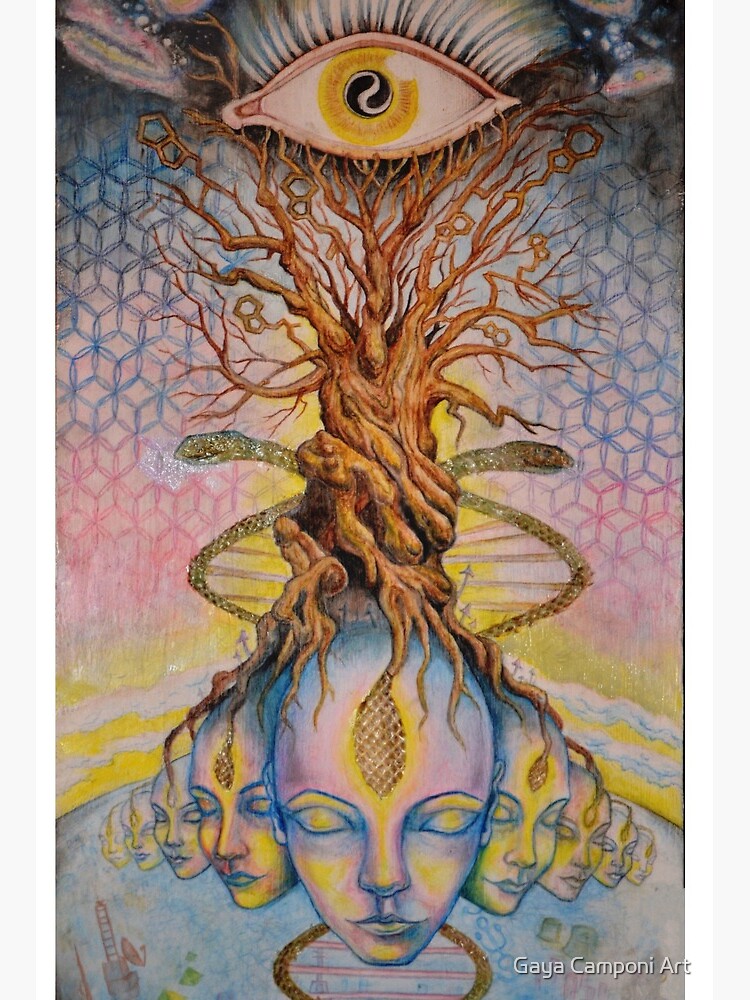The artwork, titled Gaia Camponi Art, is a mesmerizing and surreal painting featuring multiple interconnected elements. It prominently displays a giant eye at the top of the composition, which draws immediate attention. The eye has a swirling pattern in its yellow iris, with a gold area surrounding the black pupil, bordered by pink and adorned with black and pink eyelashes. Below the eye, a twisted, leafless tree emerges, with snakes branching out from the tree trunk and intertwining among its branches. The tree’s roots extend downwards, connecting to numerous identical women's faces, all bald and painted in shades of pink and blue. 

These faces form a triangle and progressively get smaller towards the edges of the painting, creating a sense of depth and distance. The central face has tree roots intricately woven into what appears to be hair, and it features yellow-colored eyes, a painted nose, and lips. The backdrop of the artwork transitions from blue, red, to yellow hues, adding a dynamic sense of movement and energy. Geometric shapes like cubes and pentagons are scattered around the sides, further contributing to the painting’s abstract and spiritualistic essence. The bottom right corner of the painting bears the signature Gaia Camponi Art in white letters, anchoring this deeply introspective piece.